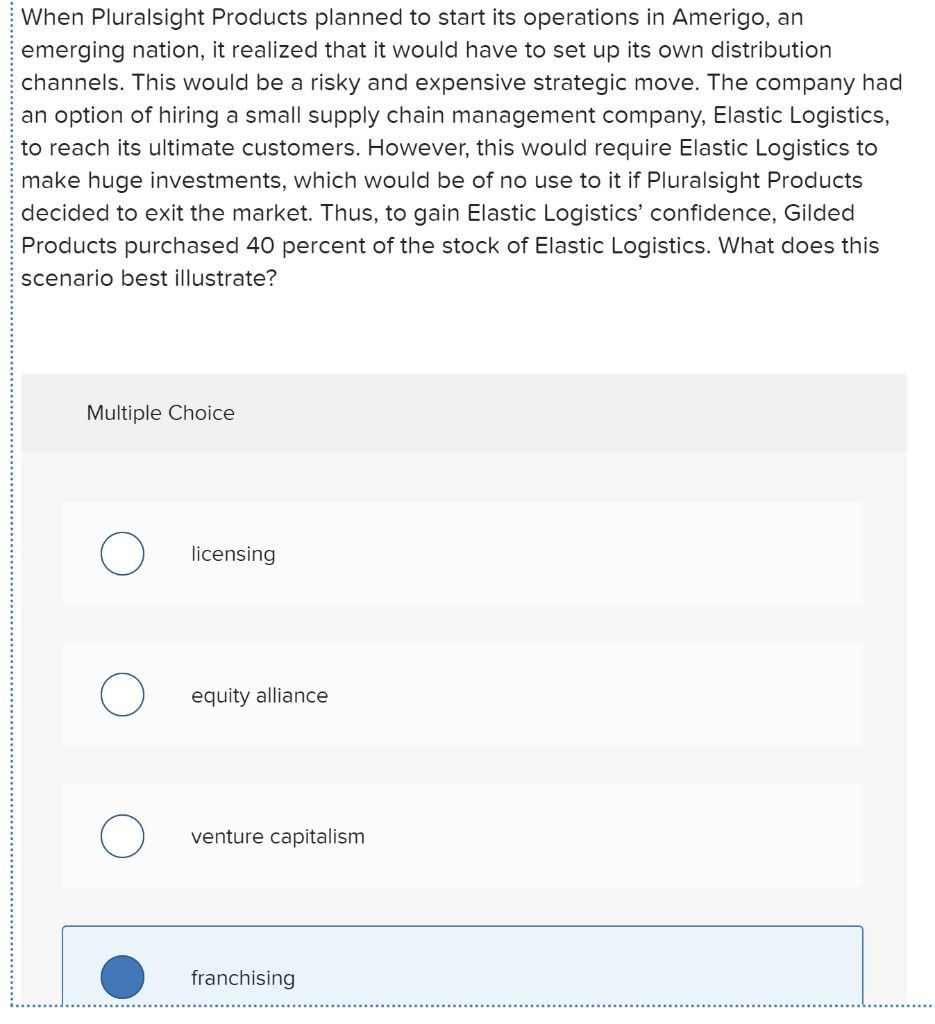This image captures a screenshot of a test question from a form or a website in portrait orientation. The background is predominantly white, featuring black text and a series of fine dotted lines. A very fine blue dotted line runs vertically down the left side of the image, with a white margin to its left, and similar dotted lines appear at the bottom.

The top of the image contains a paragraph that reads: "When Pluralsight Products planned to start its operations in Amerigo, an emerging nation, it realized that it would have to set up its own distribution channels. This would be a risky and expensive strategic move. The company had an option of hiring a small supply chain management company, Elastic Logistics, to reach its ultimate customers. However, this would require Elastic Logistics to make huge investments, which would be of no use to it if Pluralsight Products decided to exit the market. Thus, to gain Elastic Logistics' confidence, Gilded Products purchased 40% of the stock of Elastic Logistics. What does this scenario best illustrate?"

Beneath this paragraph is a gray box labeled "Multiple Choice." The gray box contains several white bars, each accompanied by radio buttons for answer selection. The multiple-choice options provided are: Licensing, Equity Alliance, Venture Capitalism, and Franchising. The "Franchising" option has been selected, causing its corresponding white circle to turn blue and displaying light blue highlighting across the bar. Additionally, a thin blue outline surrounds the selected answer choice, indicating its active selection status.